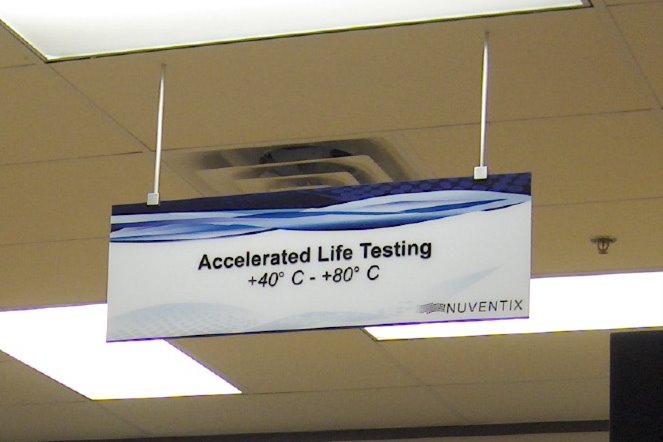This photograph captures an interior ceiling view of a building, highlighting a T-bar ceiling grid. Two distinct areas of the ceiling are brightly illuminated by overhead lights. Prominently displayed in the center of the image is a hanging sign with a white and blue color scheme. The sign reads "Accelerated Life Testing," followed by temperature ranges "+40°C and +80°C." In the bottom right-hand corner of the sign, the word "New Ventics" is also visible.